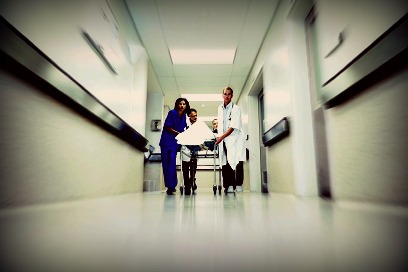The color photograph, captured from floor level, depicts a hospital hallway with a polished white tile floor that reflects the surrounding scene. In the background, a group of doctors and a nurse are seen. The doctors, clad in long white lab coats, and the nurse, dressed in blue scrubs, are collectively pushing a gurney down the corridor towards the viewer. The gurney carries a body covered with a white sheet, concealing any details of the person underneath. The hallway is sterile and unadorned, free from any signs, billboards, plants, flowers, trees, animals, or motorized vehicles. The image exudes an atmosphere of urgency and clinical sterility.